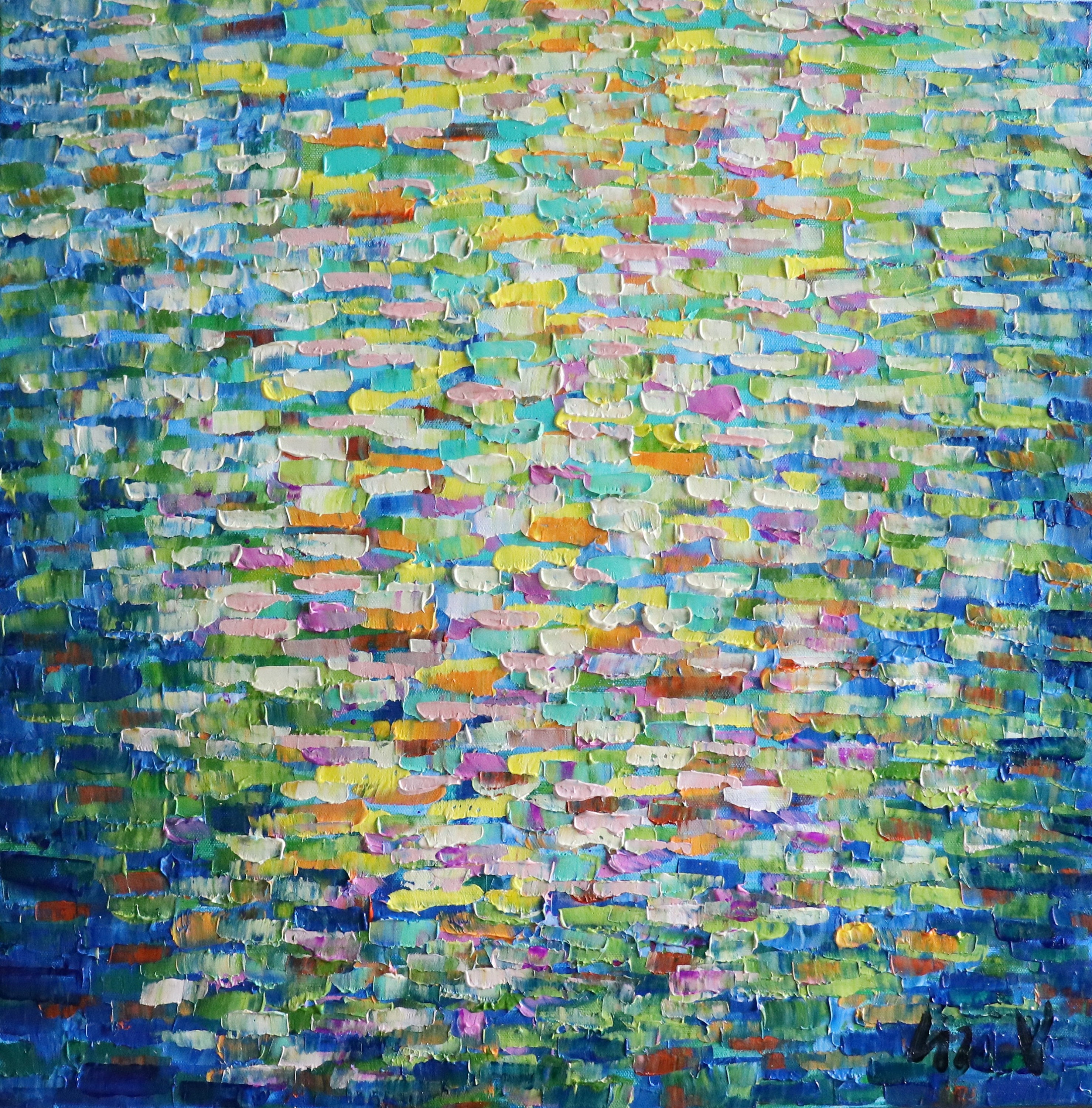The image depicts a vibrant collage composed of numerous small, rectangular pieces arranged in the style of a brick wall. The dominant color scheme transitions from dark blue at the edges, moving through shades of green and white, with the colors becoming brighter towards the center, including vivid yellows, oranges, and reds. The overall effect suggests a star or light breaking through a dark night sky. While it is unclear whether the materials used are paint or layered paper, the precise, overlapping arrangement of rectangular shapes leans towards a collage. The image features no text or figures, and at the bottom right corner, there is an indistinct signature in black ink, adding a personal touch from the artist. The image is well-lit, showcasing the colors vividly as if illuminated by natural light.